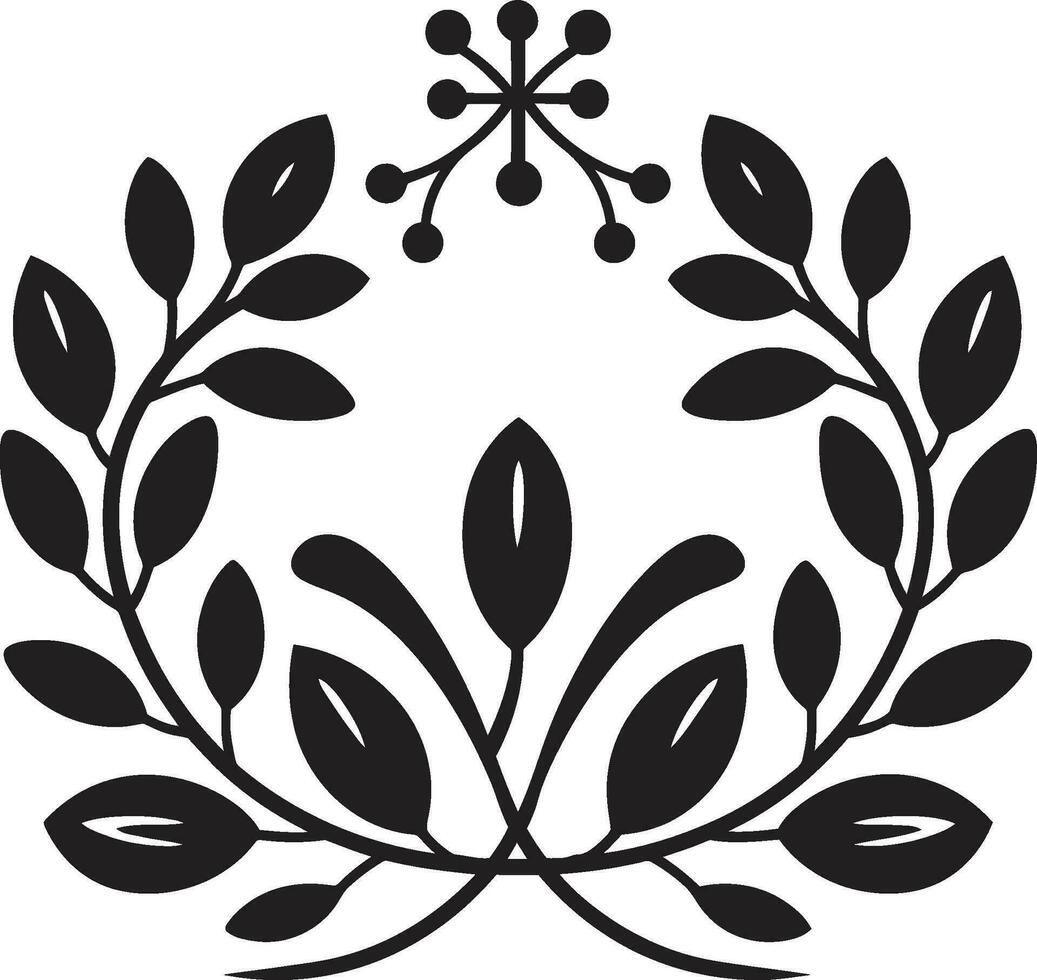The image is a simple yet artfully designed black and white drawing on a plain white background, with no definable border. The main design forms an almost circular shape reminiscent of a reef or wreath that remains open at the top. This circular pattern is adorned with numerous teardrop-shaped leaves, each shaded in black. Some of these leaves feature small white slits, adding subtle detail. At the bottom of this circle, two leaves cross over each other, forming an X. The top part of the circle, where it remains open, contains a supplementary design: a cross with diagonal lines extending from it, resembling an asterisk, each line ending with small solid black circles. The overall effect is a balanced arrangement of leaves and geometric shapes that create a visually appealing and intricate piece of black and white art.